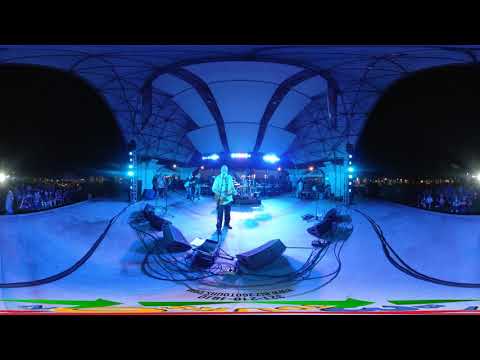The image depicts a nighttime concert scene captured from a close, on-stage perspective, giving it a slightly distorted, VR-like appearance. The stage, bathed in bluish-purple light, features a central figure—a man playing guitar and singing into a microphone—surrounded by five speakers and amplifiers arrayed in a semicircle. The back of the stage reveals additional band members, including a drum kit and various other musicians. Sitting at the stage's rear are several roadies or supporters. 

The setting is an open-air stage with an overhead structure resembling a large, white sea horn flanked by two black arches, through which the night sky is visible. Green arrows pointing to the right are prominent along the stage floor, accompanied by some illegible text. The image emphasizes the concert’s dynamic lighting and expansive open-air setup.